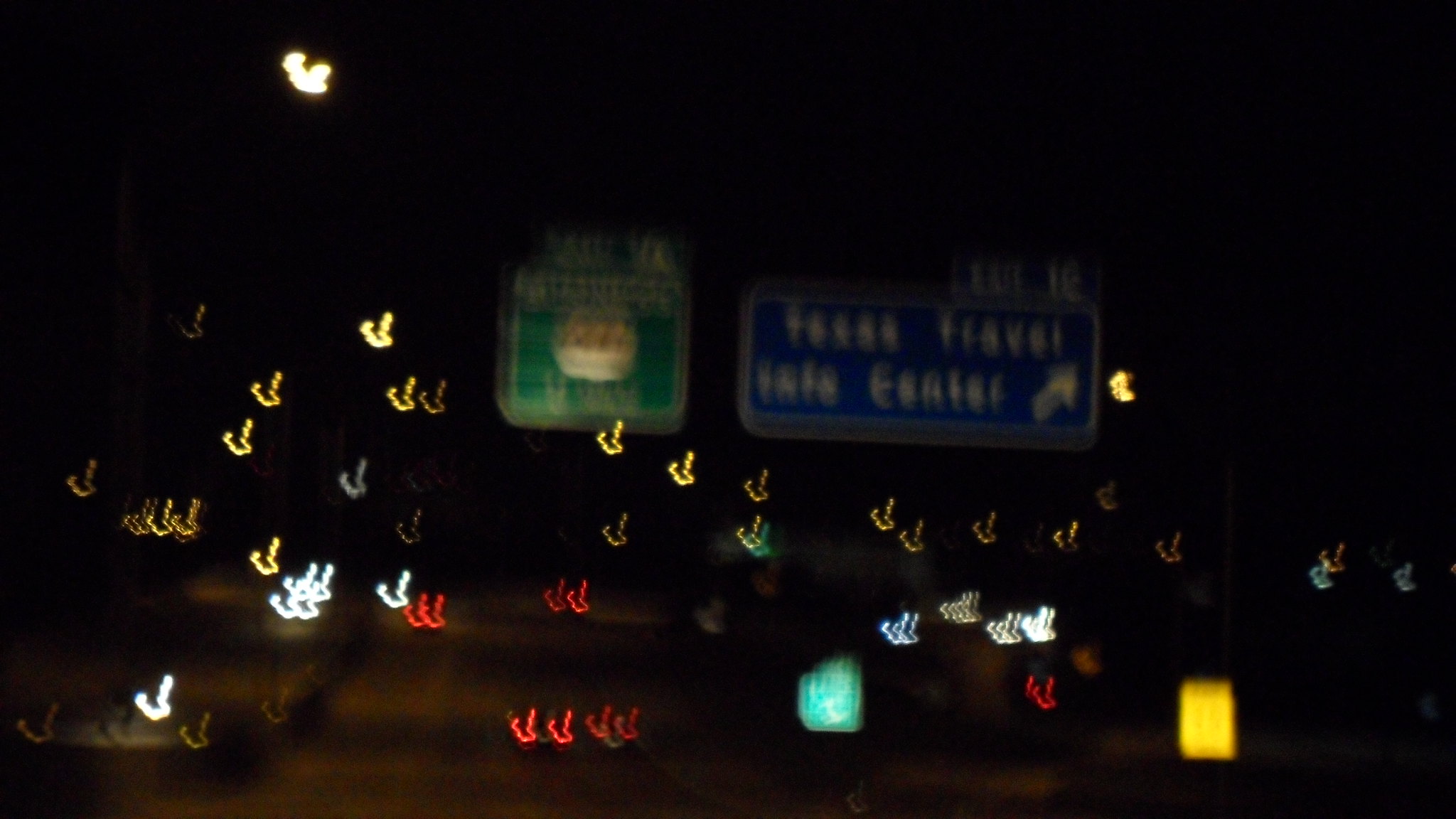The image depicted is blurry and was captured in low-light conditions. In the background, there are two noticeable signs: a square green sign on the left and a rectangular blue sign to the right. The blue sign features white text and an arrow pointing to the right. The green sign contains some text and an image in the center, which appears to be white or tan. The upper portion of the image is dark, gradually becoming slightly less dark towards the bottom. Scattered throughout the image, there are multiple V-shaped lights in various colors. Surrounding the sign, yellow V-shaped lights are prominently visible, appearing as reflections. Additionally, white and red V-shaped lights are scattered below the signs. A green and yellow rectangle is situated in the bottom right-hand corner of the image.